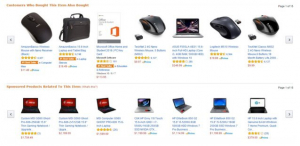The image depicts a webpage screen showcasing various tech products. At the top of the page, a gray box contains an indicator labeled "Flag as inappropriate." Several tech items are displayed, but the advertisements are blurred and unreadable. On the left side, there's a noticeable computer mouse, followed by what seems to be a briefcase and other tech items, including additional computer mice and laptops. The product descriptions are written in blue text, accompanied by gold star ratings of different quantities. At the bottom of the page, there are seven laptops displayed, featuring screens with different colors ranging from red to blue and white. Each laptop has a specific description in blue text, gold star ratings, and a price in red, although the prices are not legible.